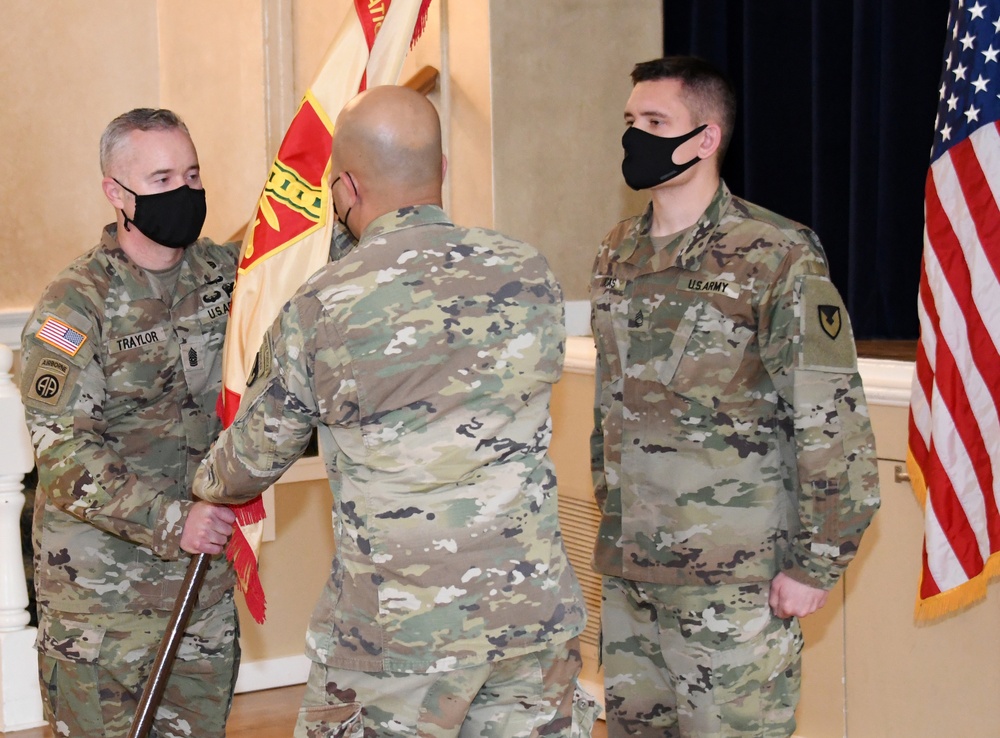In this detailed photograph, three U.S. Army soldiers are depicted in what appears to be a ceremony conducted indoors during the COVID-19 pandemic, as indicated by their dark face masks. They are clad in desert camouflage fatigues. The scene is set against a beige wall with a stage behind them, partially covered by a brown curtain. 

To the right, the room features an American flag. The soldier standing at attention to the left of the flag has a U.S. flag patch on his right shoulder. In the center, facing away from the camera, is another soldier who seems older and bald, likely an officer. He is handing over a flag to the third soldier, who stands on the far left of the image, distinguished by his black mask and short, graying hair. This flag, unlike the American flag, has a tan base with a red geometric shape in the center and possibly a horizontal chain pattern. The overall atmosphere is semi-official, indicative of a formal proceeding or presentation.